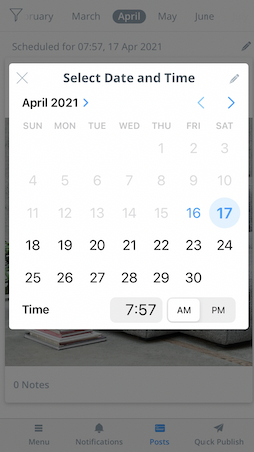A vivid and detailed image displays a digital scheduling interface prominently featuring a calendar. The foreground showcases a highlighted calendar with clear details, while a grayed-out, semi-transparent background reveals additional elements of the interface. The main focus is the interactive calendar, showing the months February through June, with a specific date, "April 17, 2021," scheduled at "7:57 AM" highlighted.

At the bottom, the interface displays four options: Menu, Notifications, Post (highlighted in blue), and Quick Publish. Above the grayed-out background, an overlay pop-up titled "Select Date and Time" appears. Within this pop-up, "April 2021" is flanked by navigational blue arrows. Below, the days of the week—Sunday through Saturday—are listed, accompanied by the dates 1 through 30. Dates 1 through 15 are in light grey, indicating their selection status. Dates 16 and 17 stand out in blue, with the 17th encircled for emphasis, and dates 18 through 30 appearing in standard black text. Finally, the scheduled time "7:57 AM" is clearly noted beneath the calendar grid.